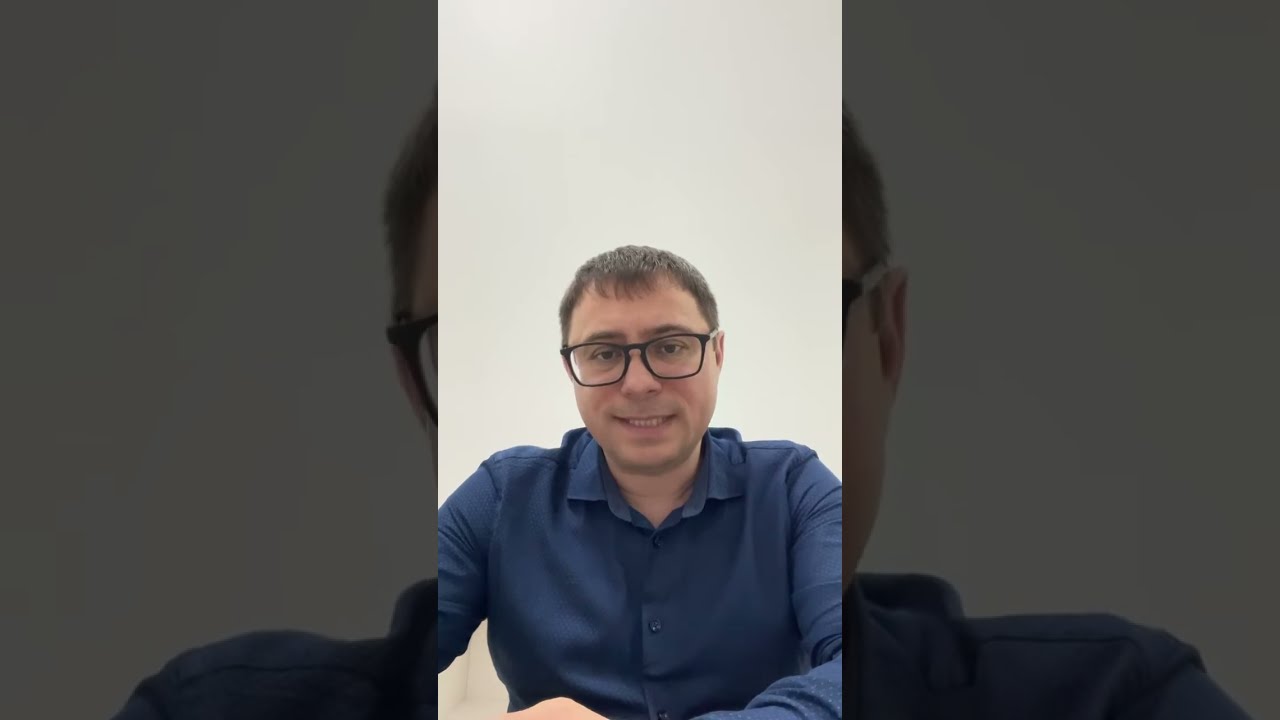This color photograph captures a Caucasian man with short brown hair, styled close to his head with a slight fringe in front. He is wearing large, black-rimmed glasses that dominate his face. His expression features a subtle grin, with his mouth slightly open, revealing his bottom teeth. The man is clad in a blue button-up dress shirt with blue buttons and a collar, and his left hand is partially visible at the bottom left of the image. The background is a plain, grayish-white, devoid of any details, enhancing the focus on him as he looks directly into the camera, reminiscent of a Zoom interview setup. The composition is primarily a portrait mode, emphasizing his upper body and face, with ample empty space above his head.